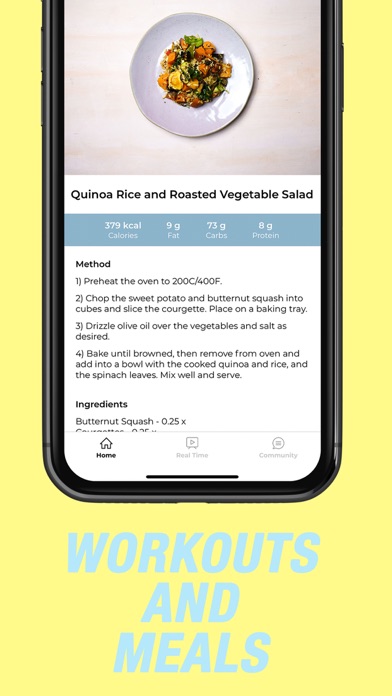The image is a screenshot of a smartphone displaying an advertisement, likely from a website. The ad showcases a recipe and is designed with a nearly square shape, slightly longer in height than in width. The background is a very light yellow hue, creating a soft and inviting look. 

At the bottom of the image, "Workouts and Meals" is written in a very light blue font, indicating the theme of the ad. Dominating the middle portion of the image is a photograph of a culinary dish, captioned in gray font as "Quinoa Rice and Roasted Vegetable Salad." A lavender-colored plate is arranged with a visually appealing assortment of roasted vegetables, including green zucchini, yellow squash, and vibrant orange carrots.

Above the photograph, there is a banner stretching horizontally in a light grayish-blue color. Below the photograph, still within the smartphone's display, is part of the recipe text on a white background, providing context and instructions related to the quinoa rice and roasted vegetable salad. The overall layout and color scheme are designed to be pleasing and easy to read, drawing attention to the healthy and appetizing meal.